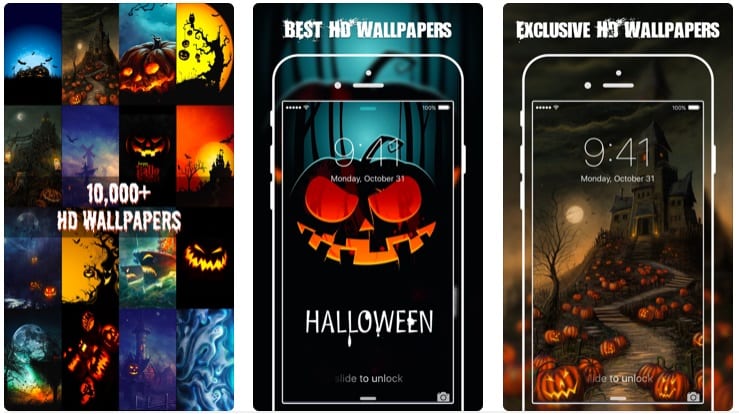The image presents three side-by-side screenshots of an online platform offering HD wallpapers for cell phones, each highlighting a Halloween theme. 

On the leftmost screenshot, there is a vertical arrangement of 16 thumbnail images, each featuring various Halloween-related designs. Among these, one can notice pumpkins, moons enveloped by eerie trees, and bats, all contributing to a spooky aesthetic. Centered amidst these thumbnails, the text "10,000+ HD Wallpapers" stands out in white.

The central screenshot prominently displays "Best HD Wallpapers" in white at the top, followed by a mock-up of a cell phone screen. The phone screen features a striking Halloween-themed wallpaper with a jack-o'-lantern at its core. The screen reads "9:41 Monday, October 31st," and "Halloween" at the bottom in white. The background fades from dark blue at the top to black at the bottom, with "Halloween" appearing to drip in white above a "Click to unlock" prompt.

The rightmost screenshot showcases "Exclusive HD Wallpapers" in white at the top, also with a cell phone outline. This wallpaper similarly displays "9:41 Monday, October 31st." The wallpaper illustrates a moonlit night scene with a winding path leading up to a haunted house. Jack-o'-lanterns line the path, casting a glowing yellow light, adding to the eerie atmosphere. This screenshot contains no additional text or images.

Each section effectively conveys an inviting, spooky ambiance perfect for Halloween, emphasizing both the variety and exclusivity of the wallpapers available.